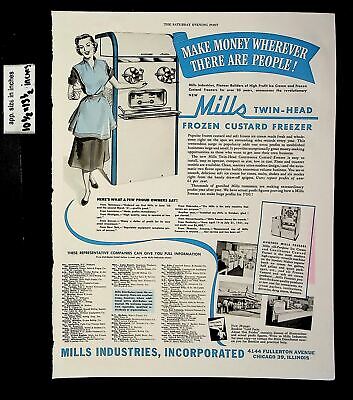The photograph captures a vintage magazine ad from the 1930s, displayed on a black table. The ad promotes the "Mills Twin Head Frozen Custard Freezer," targeted at commercial establishments like restaurants. Dominating the right side of the page is an article with text and smaller, less discernible images. 

The ad features a sketchy illustration of a stylish woman from the 20s or 30s era, wearing a blue apron over a gray skirt and black heels, standing next to a detailed depiction of a frozen custard machine. The machine is characterized by its intricate design, with circular and rectangular components, and is accented in blue.

A prominent blue banner at the top declares, "Make Money Wherever There Are People," in bold white text. Additional blue text throughout the ad includes the product name and company information: "Mills Industries Incorporated," based in Chicago, Illinois. The overall design is mostly black and white, with blue highlights enhancing key elements and a blue ribbon underscoring important features, all contributing to a visually striking and informative advertisement.